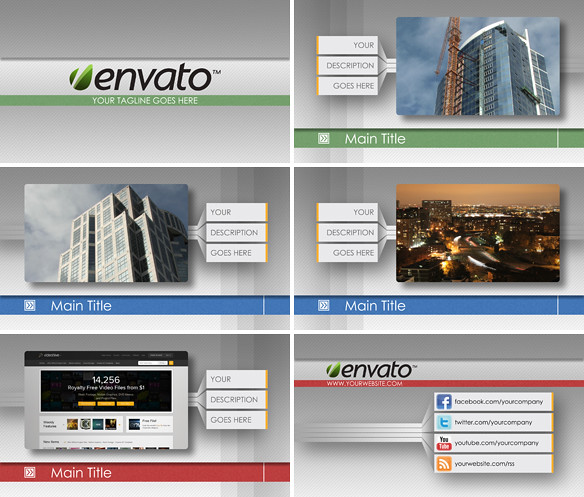The image is a website template designed for presentations, divided into six sections with a focus on showcasing Envato as an example company. Each section is in shades of grey, with key elements highlighted in green, blue, and red. 

The top left section features the Envato name and a placeholder tagline, with the text "your tagline goes here." The top right section contains an image of a building alongside the text "your description goes here," and a "main title" at the bottom. 

In the middle left section, another building is depicted with the accompanying text "your description goes here," followed by a "main title" below. The middle right section offers an aerial view of a city with similar text and a "main title" at the bottom.

The bottom left section presents a screenshot of a website with the text "your description goes here" to the right and a "main title" in a red color band at the bottom. The bottom right section lists social media platforms—Facebook, Twitter, YouTube, along with a placeholder for "your website." The top left of this section repeats the Envato name.

This template aims to provide companies with a clear preview of how their websites could look using Envato’s design service, featuring internet technology-oriented elements and placeholders for essential information and links.